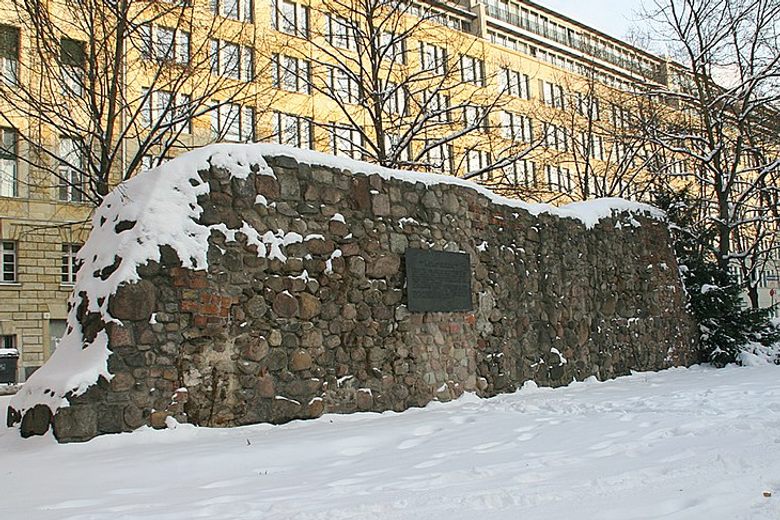The photograph showcases a vast and imposing yellow brick building, approximately six to eight stories high, stretching beyond the frame on both the left and right. The facade is dotted with numerous windows and appears to have penthouse-style rooms with balconies on the uppermost levels. In the foreground, a historic stone wall, constructed from a mix of round and square weathered rocks, stands prominently. The wall, partially covered in three to four inches of snow, is visibly aged and slightly dilapidated, with some stones having fallen off over time. A dark metal plaque, presumably of historical significance but unreadable in the photo, is affixed to the wall. The area in front of the wall is blanketed in snow, crisscrossed with footprints and paths. Leafless trees, stark against the winter backdrop, line up behind the wall while a solitary pine tree stands tall on the right. The overall scene evokes a sense of historical significance and the quiet stillness of winter.